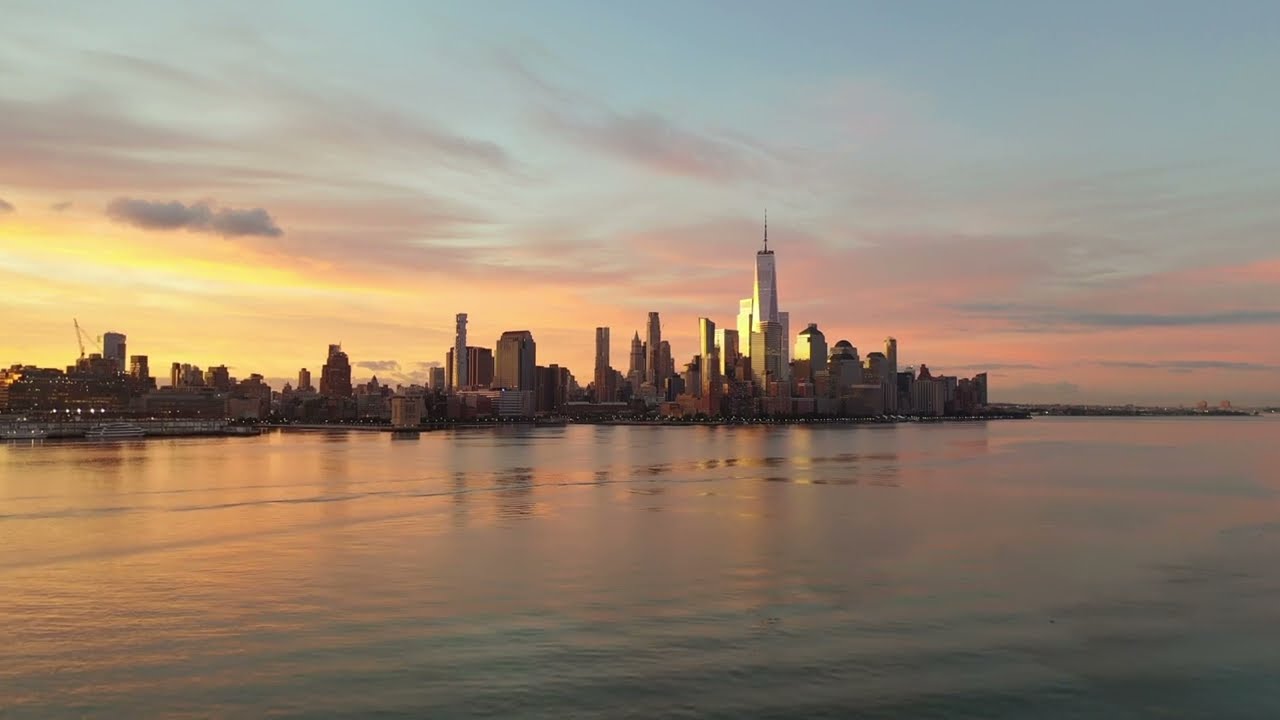This stunning evening cityscape captures a tranquil urban skyline against the calm ocean, with a gentle mist hovering above the water’s surface. Dominating the center is an imposing skyscraper with a sharp point, towering above surrounding buildings. Progressing to the right, the skyscrapers gradually diminish in height until they reach the city's edge. To the left, another cluster of tall, sporadically placed buildings is visible, tapering off into shorter structures, with a distant construction crane marking the skyline far in the left background.

The sky is partially clouded, painted in hues of pink and yellow from the setting sun, which creates a striking play of colors that fade to bright yellow on the left side. The scene, possibly viewed from an opposing island or a boat, features the city's reflections shimmering on the water, with buildings in varying shades of beige, white, and black. A barge-type ship is docked to the left, adding to the bustling yet serene maritime tableau.

As dusk approaches, the scene evokes the timeless charm of a postcard, reminiscent of iconic views like New York City from a distance, with Manhattan's skyscrapers rising above the calm water. The peaceful ripples on the ocean and the picturesque sunset enhance the image's beauty, making it a captivating visual narrative.